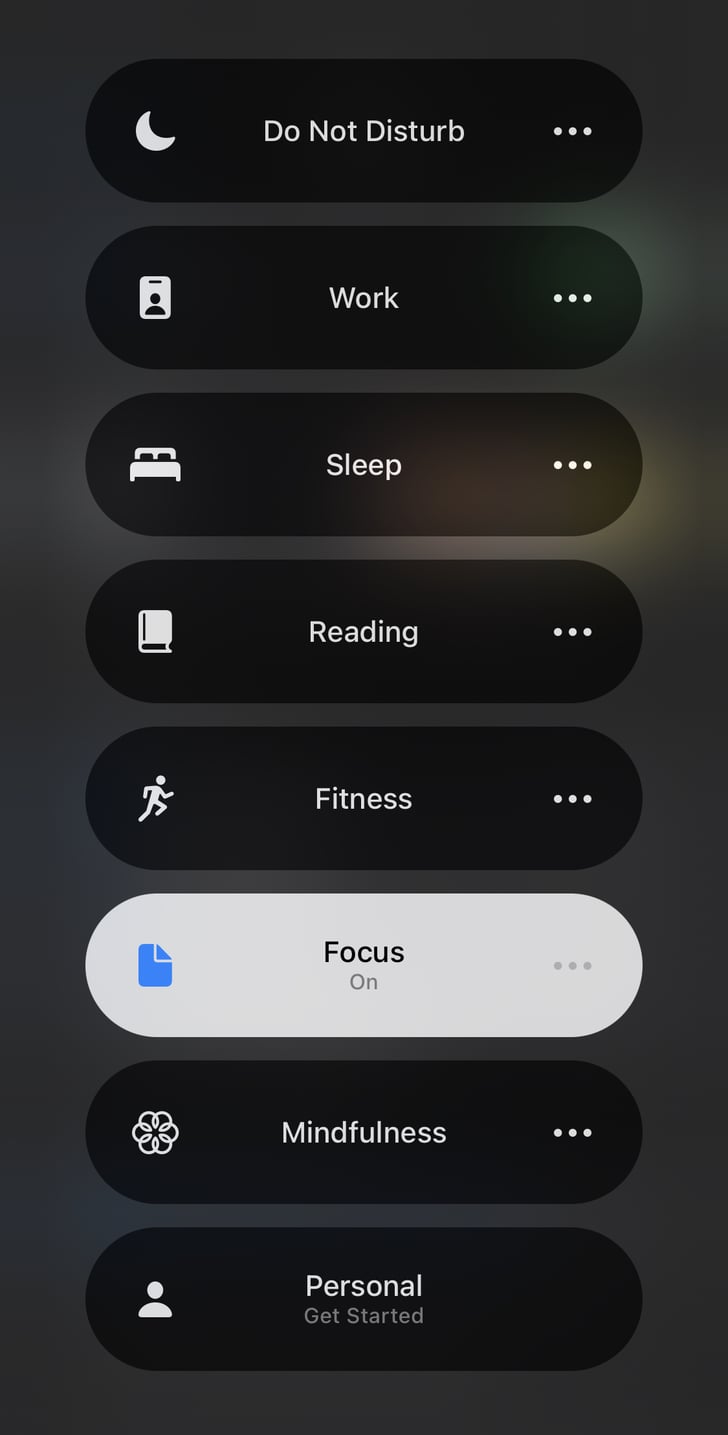The image showcases a series of eight shortcut buttons, each with a transparent black background and white text. The buttons feature a uniform layout, with icons on the left side and all text in white, except for one highlighted entry. Each button has a three-dot horizontal menu option on the right side, except for the last button, which lacks this feature.

1. **Do Not Disturb:** At the top, this shortcut is accompanied by a moon icon on the left.
2. **Work:** This option features a name tag icon on the left side.
3. **Sleep:** Represented by a bed icon located to the left.
4. **Reading:** A book icon is placed on the left side of this shortcut.
5. **Fitness:** Displayed with a running figure icon on the left.
6. **Focus:** This entry stands out as it is highlighted in white, with the text in black. A blue picture frame icon is on the left.
7. **Mindfulness:** Accompanied by a white icon on the left.
8. **Personal:** Below the label, it says "Get Started." It has a profile icon positioned to the left.

All icons are rendered in white, maintaining a consistent appearance across the panel while differing only in the icon's imagery.